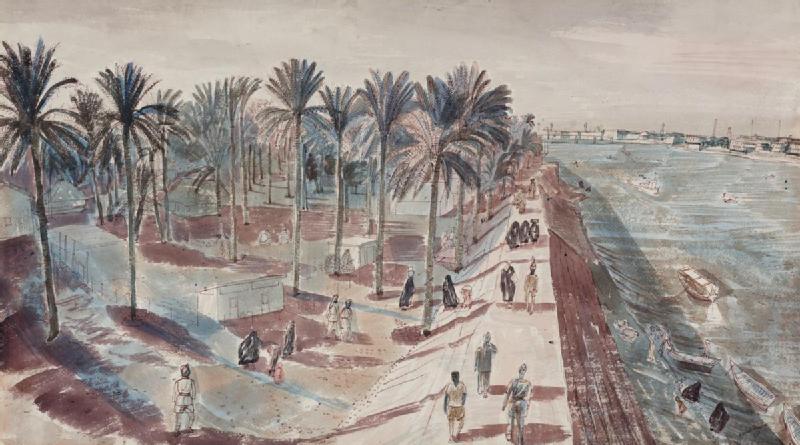The image depicts a faded, horizontal rectangular painting or drawing dominated by subdued hues of beige, gray, brown, and dark green. The left side features a cluster of palm trees or coconut trees with thin, grayish stalks and dark green, almost black foliage. Below the trees, patches of barren soil interspersed with minimal grass cover the ground. 

Moving to the right, a beige, elevated seawall stretches vertically from the bottom to about two-thirds up the image, bordering a light blue body of water. The water, dotted with indistinct floating objects and a few rocks and boats, separates the seawall from a cityscape visible in the background, comprising low, white buildings.

The walkway atop the seawall is populated by people; men dressed in shorts and T-shirts or shirts and pants, and women in dark burqas, hinting at a possible Muslim country. To the left of this walkway, an open brown field with scattered small white buildings can be seen, also populated by a few individuals. The entire scene is set against a pale, grayish-beige sky, lending a stale, drab ambiance to the picture.